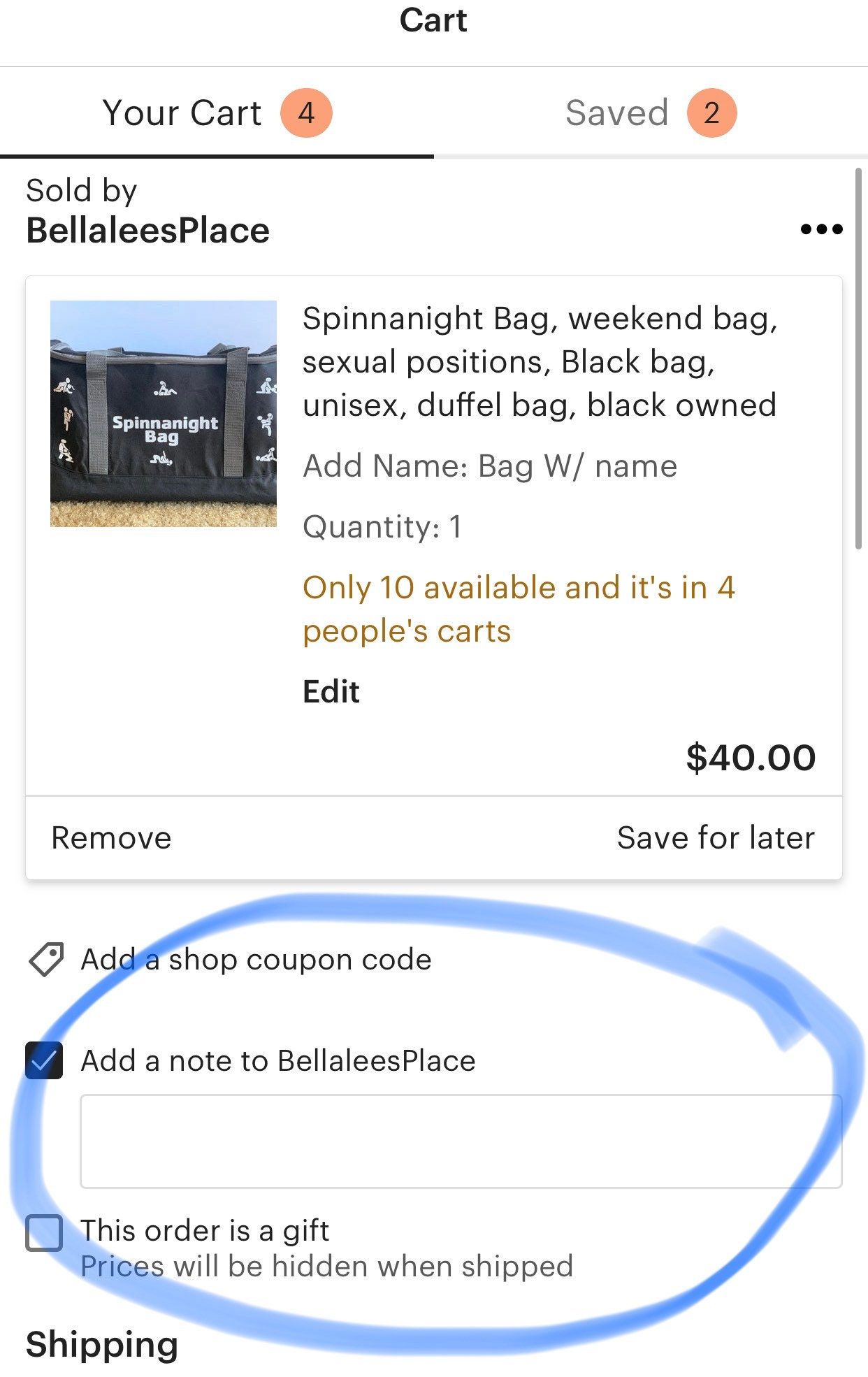The image captures a shopping cart interface from an online store. At the top, the word "Cart" is prominently displayed, centered at the top of the display. The cart contains four items, with two additional items saved for later. The products are sold by "Bella Lee's Place."

One featured product in the cart is a black duffel bag adorned with white prints of generic figures in various exercise positions. The bag has gray handles and is marketed as a "Spin-a-Night Bag," suitable as a weekend or a unisex duffel bag. It is noted for being a creation of a black-owned business. The product listing highlights that only 10 bags are available, and it is already in four other people's carts. This bag is priced at $40.

The interface provides options such as removing the item, saving it for later, adding a shop coupon, and marking it as a gift. Notably, the "Add a note to Bella's Place" option is emphasized with a large, light blue marker-like circle, indicating its importance. This option has been checked by the user, suggesting they have opted to include a personalized note with their order.